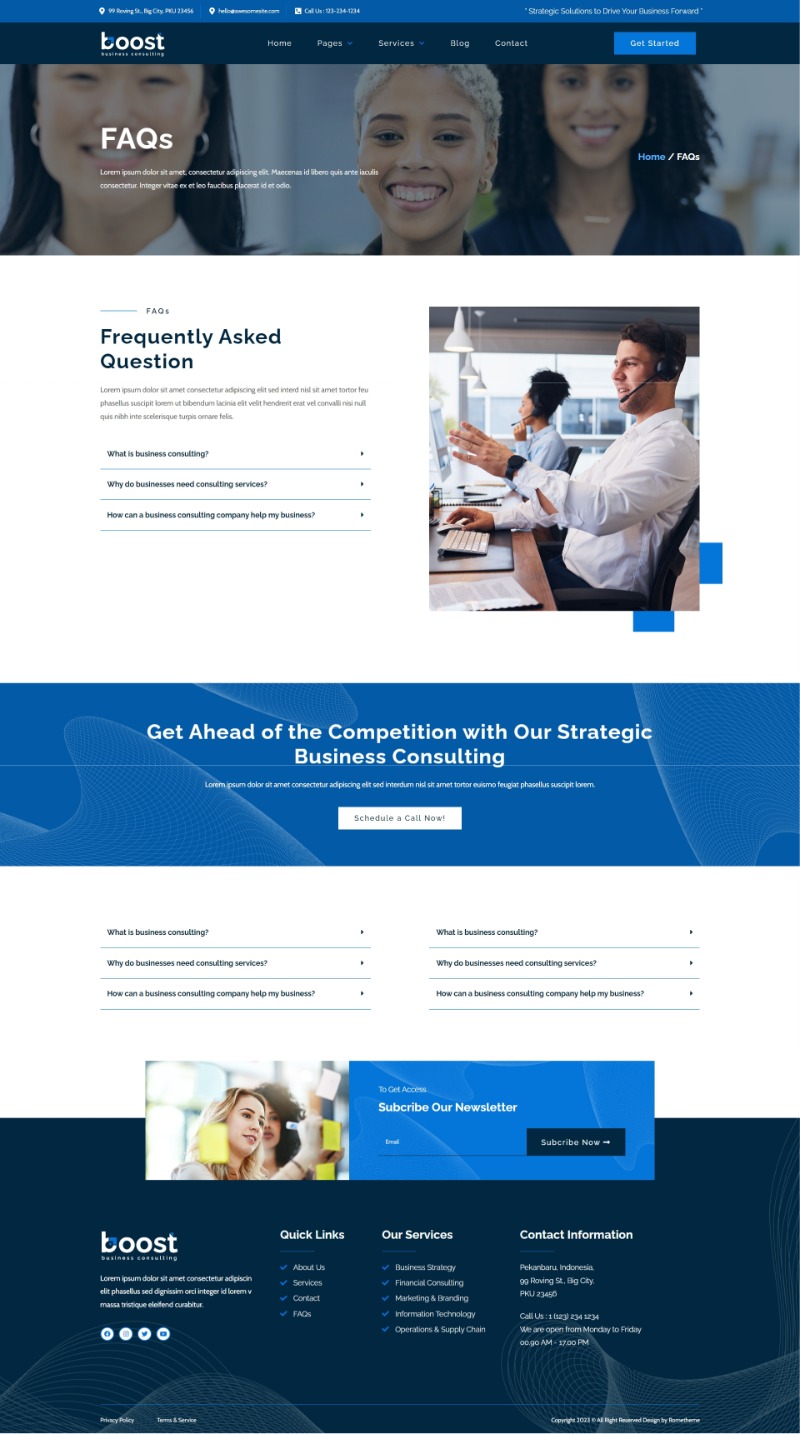The website for Boost features a clean and professional design. At the top of the page, a blue banner spans the width of the screen, displaying a vibrant photo of three smiling women facing the camera. The company name, "Boost," is prominently displayed in white type over the photo, while the navigation menu is arranged neatly across the top with links to Home, Pages, Services, Blog, Contact, and Get Started.

Overlaying the picture of the three women, the word "FAQS" is displayed. Beneath this banner, there is a white section of the page where a comprehensive FAQ section begins. It includes text in a foreign language followed by a detailed explanation in English: "What is Business Consulting? Why do businesses need consulting services? How can a business consulting company help my business?"

On the far right side of the page, another image shows two people—a woman and a man—both wearing headphones with mouthpieces, intently focused on a computer screen. Below this image, a blue rectangular box contains the text “Get ahead of the competition with our strategic business consulting,” followed by another line in a foreign language and the call-to-action, “Schedule a Call Now.”

At the footer of the page, the FAQs are reiterated: "What is Business Consulting? Why do businesses need consulting services? How can a business consulting company help my business?" Additionally, there's a photo of two women engrossed in their work, with one of them writing something on a piece of paper. The page invites visitors to subscribe to their newsletter with the message, "To get access, subscribe to our newsletter."

Overall, the website offers a user-friendly interface with strategically placed images and informative text, designed to assist visitors in understanding the benefits of business consulting and encouraging them to take action.